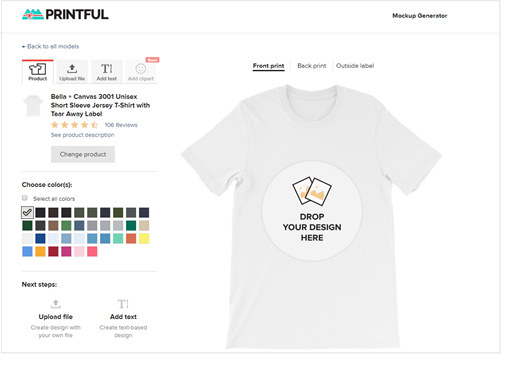The webpage displayed is from Printful, a custom clothing platform that allows users to design their own t-shirts. The company's logo, located in the upper left corner, features the name 'Printful' alongside three green mountain peaks with a red bar across them. In the upper right side of the screen, the text "Mockup Generator" is prominently displayed, indicating the core function of the page. The left sidebar contains a wide array of customization options, enabling users to choose the t-shirt color, upload designs, add text, and switch between different types of apparel, such as short sleeve and long sleeve shirts. Overall, there are approximately 40 different customization options listed. The right side of the screen showcases a mock-up of the t-shirt, which is currently plain white with a designated area in the center instructing users to "drop your design here."